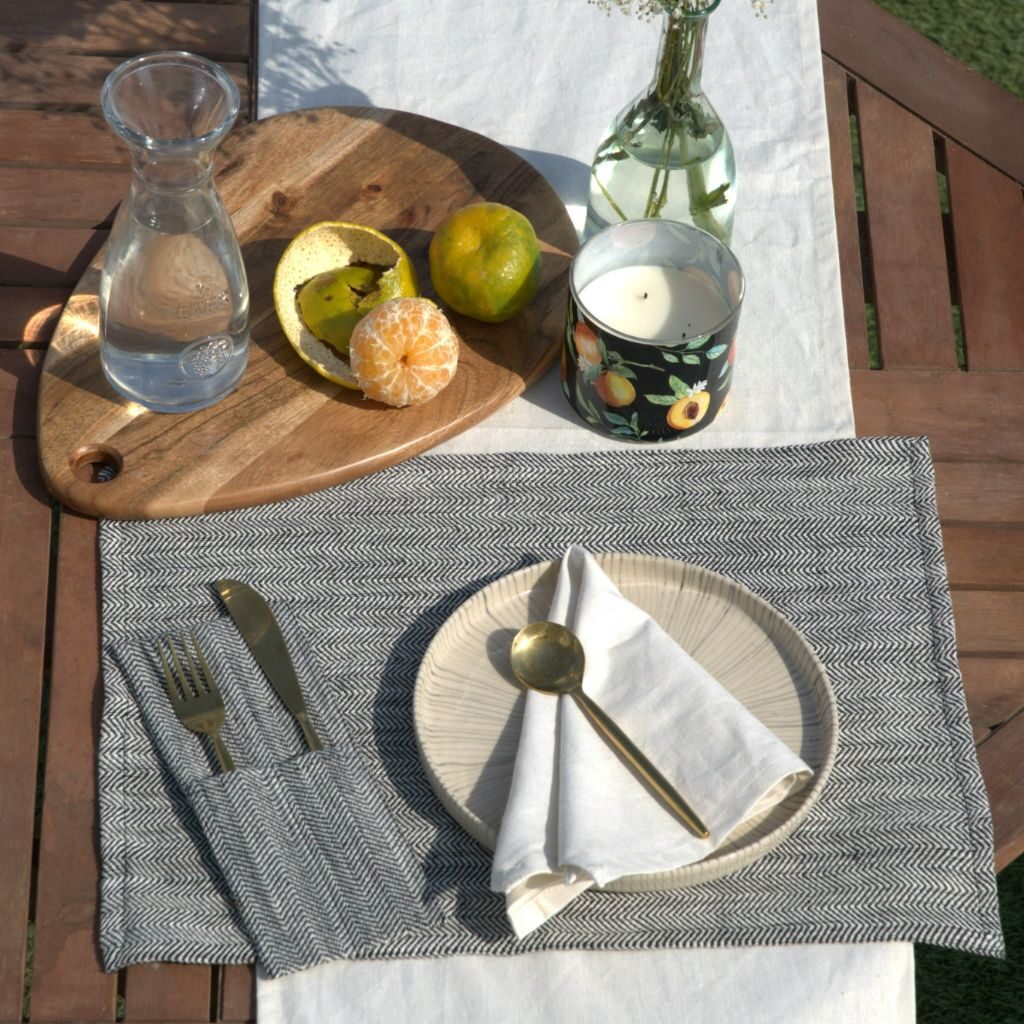This large, square picture captures an inviting outdoor table setting bathed in sunlight, with visible greenery through the wooden slats and in the background. The wooden table, characterized by its darker tone, features a pristine white runner laid vertically. At the center, a setting includes a gray and black chevron-patterned placemat with a matching napkin holder containing a knife and fork. A small, tan-patterned plate, adorned with a folded white napkin, supports an antique-looking golden soup spoon. Adjacent to this arrangement is a wooden cutting board, shaped like a guitar pick, holding a carafe of water, a peeled citrus fruit, and a pear. A candle with a black fruit pattern, unlit, and a vase filled with water and flower stems, though cut off from view, add to the artistic composition. The scene is completed by the thoughtful placement of these items on the runner, creating an aesthetically pleasing and inviting atmosphere despite the simplicity of the food and drink present.